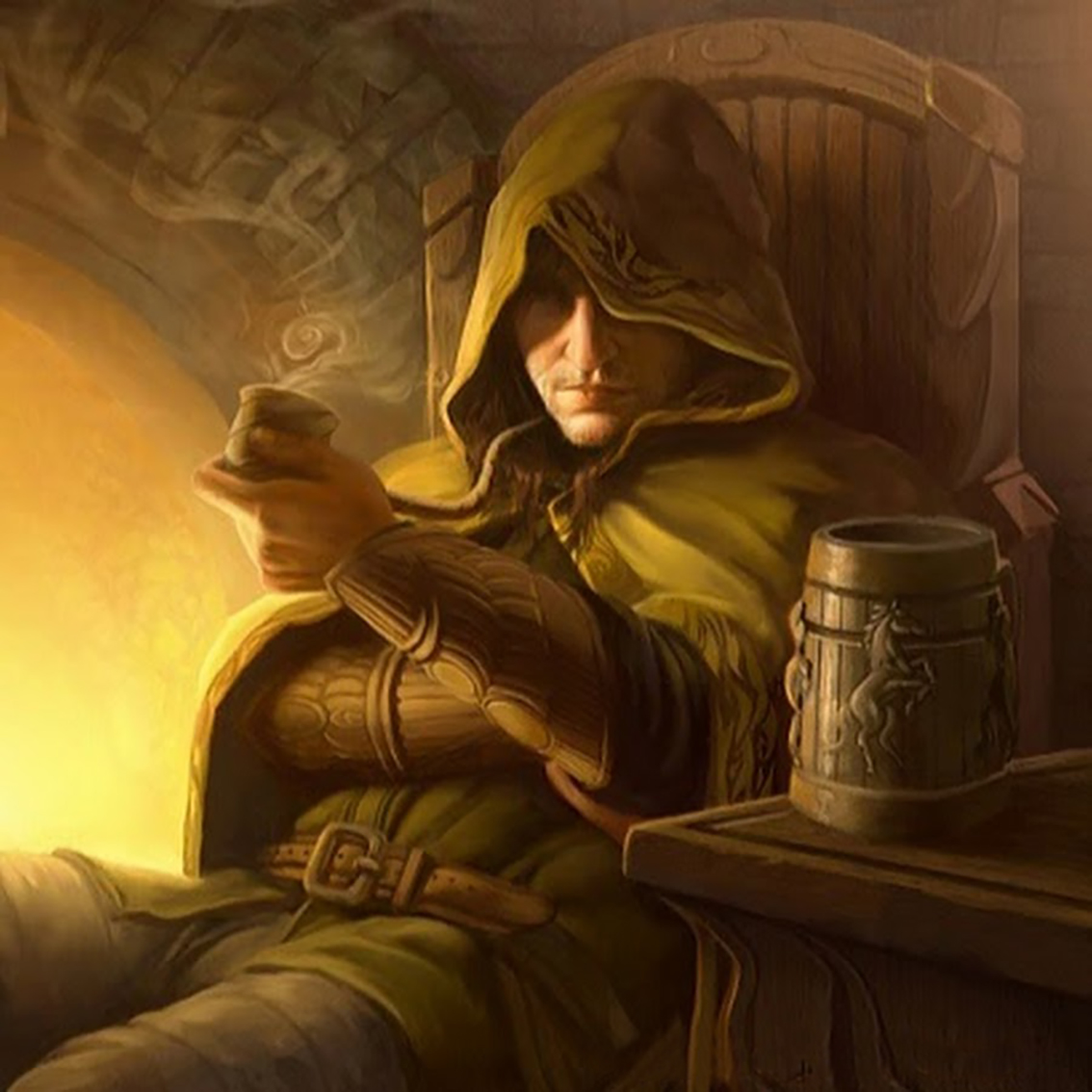The illustration depicts a serene medieval or fantasy setting, featuring a cloaked man seated in a tall, wooden chair by a fireplace. The predominantly brown, beige, and yellow-toned scene exudes warmth and coziness. He is dressed in a green shirt with a brown leather belt and rust-colored gauntlets covering his forearms. His hooded cloak casts a shadow over his face, leaving only his nose and mouth visible. In his left hand, he holds a steaming cup, while his right hand rests casually. Next to him, on a wooden table, stands a large, ornate mug with carved images of rearing horses, indicative of a bygone era. The glow from the fireplace reflects golden hues, adding to the overall mystical and old-world charm of the room, reminiscent of something out of a fantasy RPG or a scene from "The Lord of the Rings."